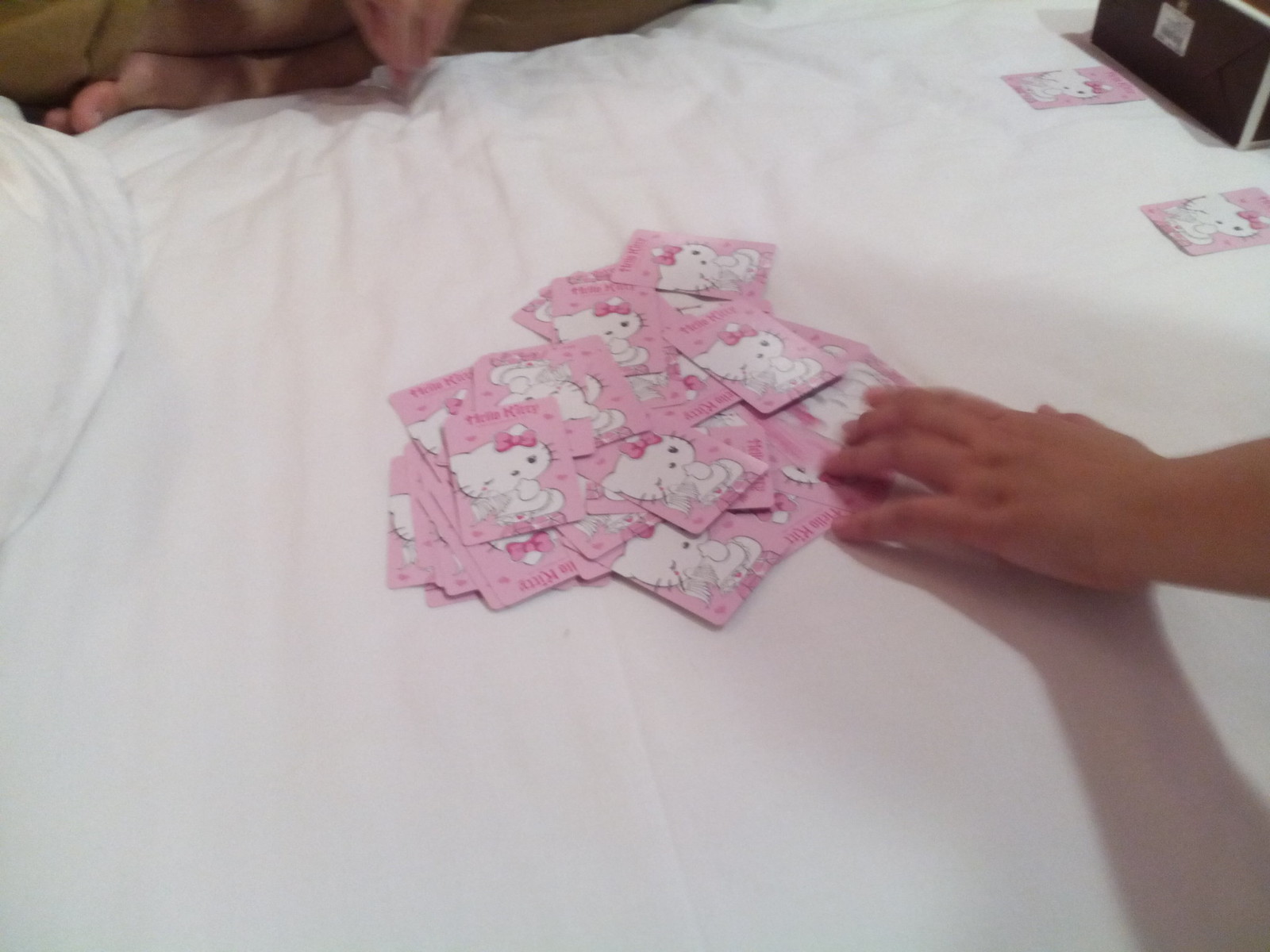The image features a scattered pile of Hello Kitty playing cards placed on top of a white blanket, likely on a bed. In the center-right of the image, a left hand reaches out, positioned at the bottom part of the card pile. In the upper left corner, another person is sitting cross-legged, with their legs, a foot, and a slightly blurred hand, with one finger touching the bed, visible. The image also includes a snippet of a white pillow on the left-center side. In the upper right corner of the image, two Hello Kitty playing cards are prominently displayed, mostly pink with an illustration of a white kitten adorned with a pink bow on the upper left corner of its head. Behind these two cards, a black box is partially visible.